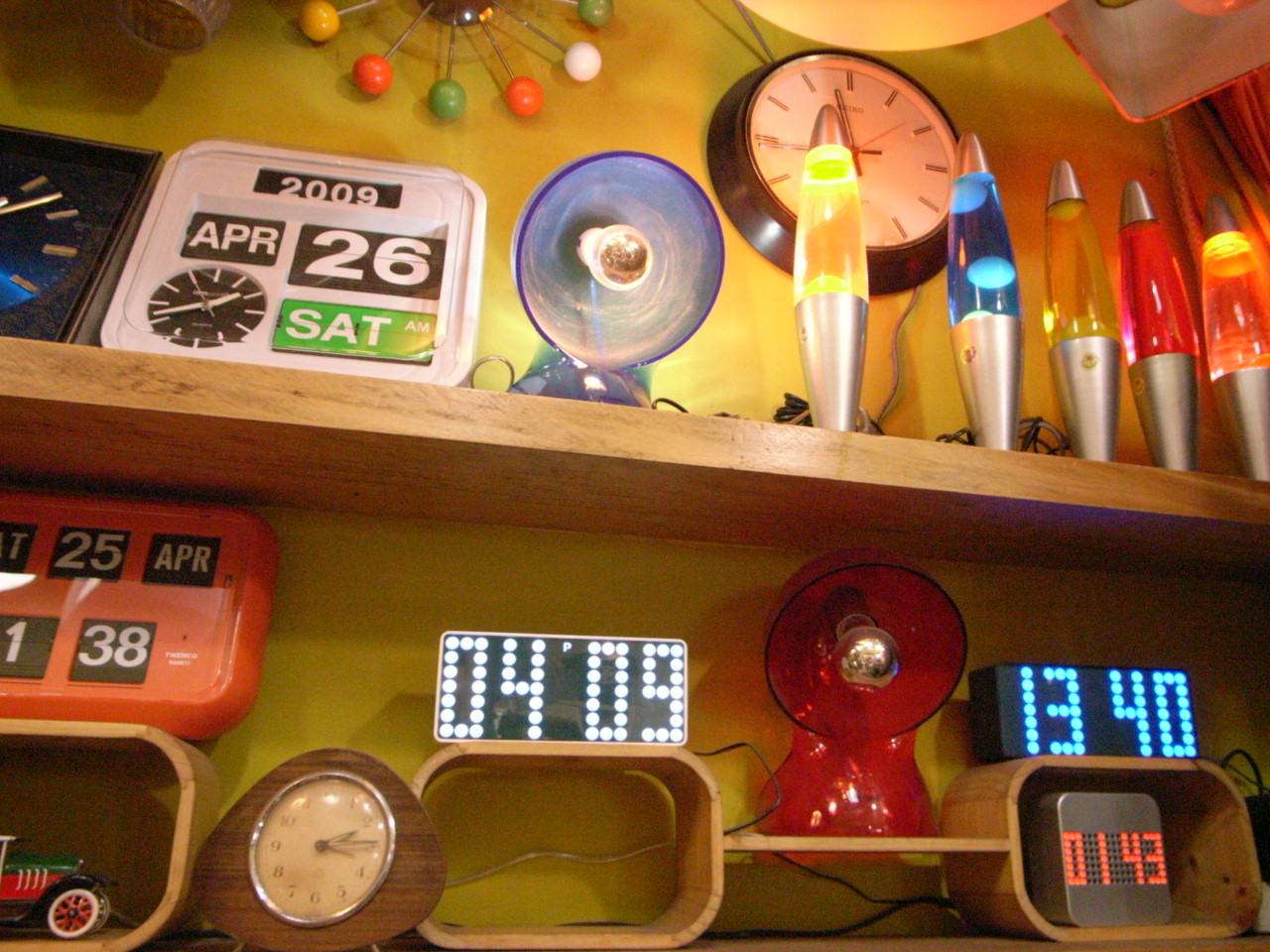This is a vibrant and detailed color photograph taken indoors under artificial lighting, featuring two shelves brimming with an eclectic assortment of decorative objects. The top shelf prominently displays several intriguing items: starting with a black sign boldly displaying "1009" atop two smaller black squares labeled "April" and "26." Next to this arrangement is a round clock with a black face and contrasting white hands, situated beside a green square displaying a simple white inscription. Dominating the center is an enigmatic object resembling either a giant soother or a satellite dish, its exterior painted blue and inner surface white.

In the background, a wall clock is visible. Just below it, neatly lined up, are five metallic-bottomed lava lamps in a sequence of colors: yellow, blue, yellow, red, and red. Mounted above these lava lamps is a uniquely designed decorative clock, featuring an array of ping pong balls in yellow, red, green, and white.

The lower shelf showcases an impressive variety of decorative clocks. This collection includes clocks with digital displays and others with traditional round faces, as well as an unusual model without a display, only featuring two hands enclosed within a square frame. On the far left sits a distinctive orange clock, bearing a striking resemblance to the white square clock positioned above, creating a sense of thematic continuity within the display.